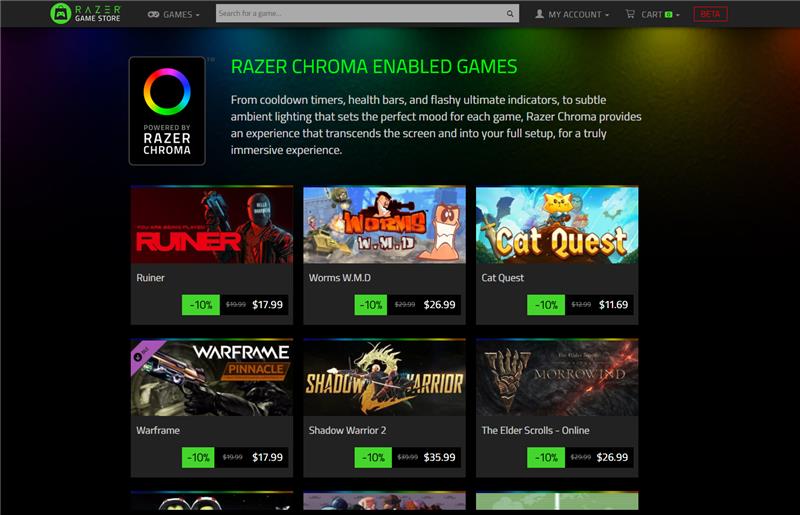This image features a screenshot of the Razer Game Store website. At the very top of the image, a gray bar stretches across the width of the screen. In the upper left corner of this bar, the Razer logo is displayed in green, accompanied by a green and black shopping bag icon with "Game Store" written in white beside it. 

To the right of this, there is a drop-down menu labeled "Games." Centrally positioned within the gray bar is a large white search bar. On the far right, options for "My Account" and "Cart" are available. 

Beneath this top navigation bar, the background features a combination of colors, including shades of blue, teal, lime green, yellow, and red. These colors appear as blurred light streaks shining from the top. 

Centrally, the text "Razer Chroma Enabled Games" is prominently displayed, followed by information about these Chroma-enabled games. Below this information, various game cover arts are arranged in tiles. 

The visible tiles showcase six games: "Ruiner," "Worms," and "Cat Quest" at the top, followed by "Warframe," "Pinnacle," "Shadow Warrior 2," and "The Elder Scrolls Online" at the bottom. Additionally, three more game tiles are partially visible at the very bottom but are cut off from view.